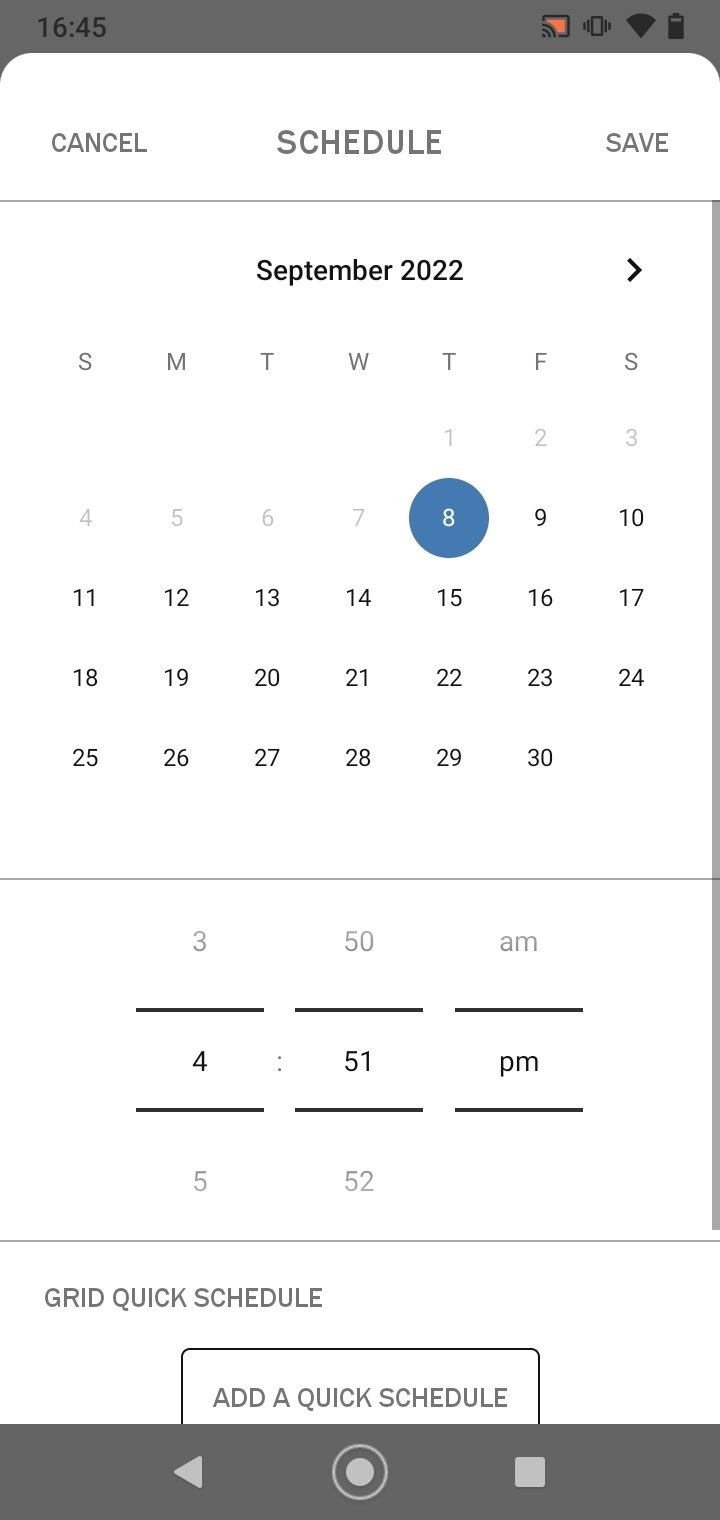The image is a screenshot captured from a cell phone. At the top of the screen, a dark gray header displays black text indicating the time as "16:45" in the upper left corner, while the upper right corner features black icons for Wi-Fi and battery status. Beneath the header, a calendar for September 2022 is shown on a solid white background.

In the upper left, small gray text reads "Cancel," centrally placed bold text states "Schedule," and the upper right corner shows "Save," all aligned above a thin gray horizontal line. Below this line, the September 2022 calendar is displayed with a blue circle around the date September 8th, emphasizing this day. Another thin horizontal gray line separates the calendar from the subsequent information, which lists "3:50 AM" and "4:51 PM" below.